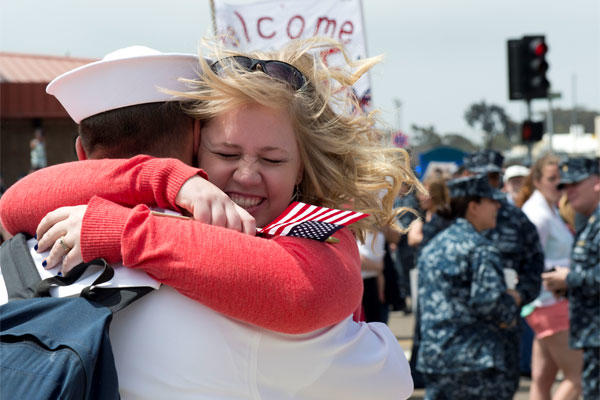The image depicts a heartfelt military homecoming scene. In the foreground, a woman, with blonde hair and donning black glasses on her head, embraces a sailor. The sailor, dressed in a traditional white uniform and hat, has a blue backpack with black straps and is looking away from the camera. The woman's eyes are closed as she smiles, revealing her teeth, and she holds a small American flag in her right hand. 

In the background, there is a large white banner with the word "Welcome" written in red prominently displayed. A stoplight showing red is visible on the upper right, and various individuals clad in military fatigues are on the right side of the frame. One woman in the background is wearing pink shorts and a white shirt. The scene is accentuated by a multitude of colors, including the red roof and gray facade of a building to the left, green trees underneath the stoplight, and scattered hues of blue, peach, and orange, particularly evident in a structure seen in the upper left of the image. This collective imagery vividly captures the joy and emotion of a military homecoming, with the central focus being the woman's touching reunion with the sailor.